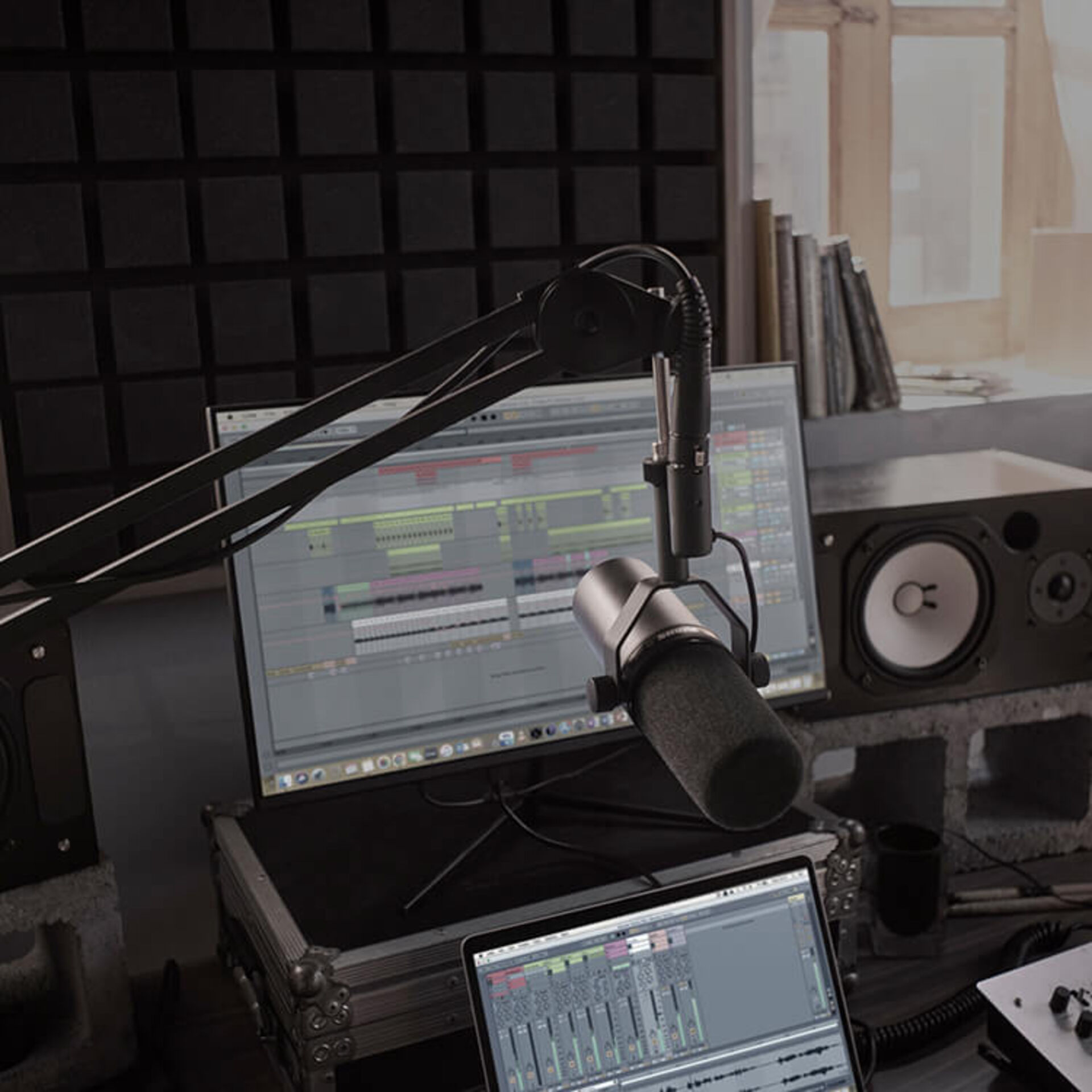The image depicts a detailed setup for a home DJ booth or portable radio station. Central to the setup is a professional black microphone positioned prominently in front of a computer monitor displaying audio settings. Adjacent to the monitor is a partially visible tablet encased in a protective black case with aluminum trim. Flanking the setup are two large black speakers, each sitting on cinder blocks for stability. Beneath the main computer monitor, a portion of another screen or laptop can be seen. 

The backdrop features a black checkered foam wall, likely for sound insulation, with sound insulation material framed in front of the booth for additional noise control. To the right of the setup, a double glass door leads to another space, and in front of this door is a shelf or window seat holding several books, giving a more personal, home-like touch to the studio. The equipment appears highly portable, suggesting that the entire setup could be easily packed up and transported if needed.